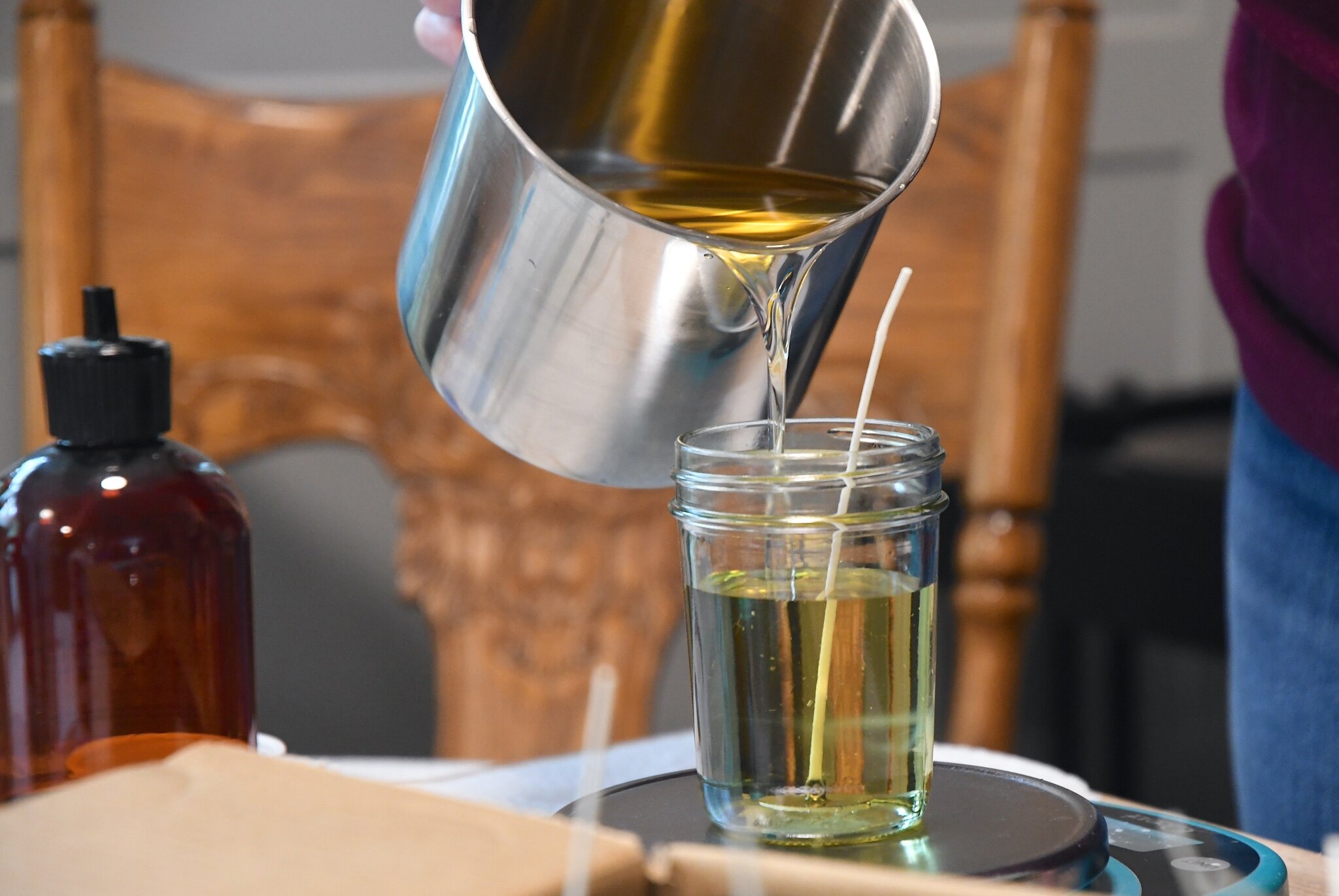In this detailed image, a person clad in a red (or burgundy) sweater and blue jeans is partially visible, pouring a light green or olive oil-colored liquid from a large metallic stainless-steel pitcher into a glass mason jar. The jar, which is about three-quarters full, has what appears to be a wick inside, suggesting that the scene depicts candle-making. The mason jar is placed on a round, flat, black surface, likely part of a scale given the teal green base beneath it that appears to have buttons. Adjacent to the jar, on the table, there is an amber-colored squeeze bottle with a black cap, and an open brown cardboard box lies at the bottom of the image. The background is out of focus, showing what seems to be a dining room chair.